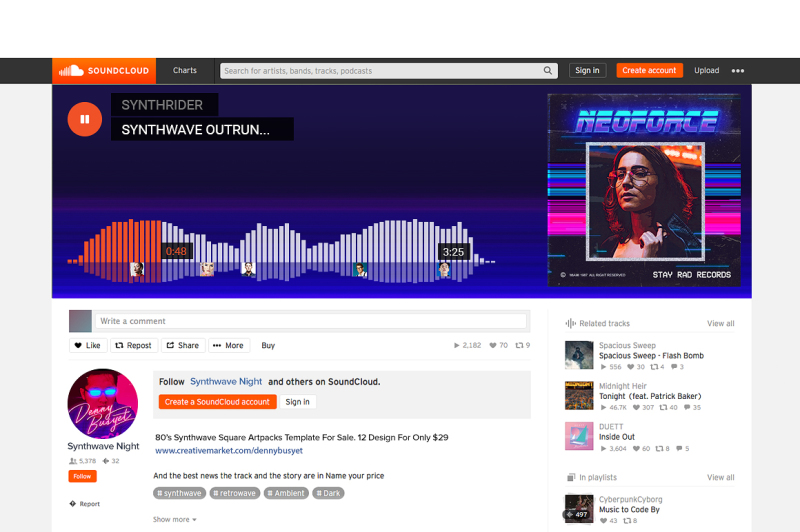The image captures a detailed interface of a SoundCloud page featuring a music track. At the top, there's a vibrant orange rectangle with the SoundCloud logo, including an icon of a cloud. Below that, a search box with a magnifying glass icon is positioned alongside options for signing in, creating an account, and uploading content.

Centered prominently is a music player interface. A red button with a pause symbol is featured, suggesting the current playback status. The track title "Synth Rider" is displayed, followed by "Synthwave Outrun..." Below the title, on the right side, an album cover is shown. It features a woman wearing glasses, illuminated by a red light that highlights her hair, and surrounded by multicolored stripes. The album name "Neo Force" is styled in a spacey, italic font.

To the left of the album cover, an audio waveform is visible, mostly white with a red section at the beginning, indicating the playback progress. Scattered along the waveform are tiny thumbnail pictures of various people, possibly indicating listener interactions or comments at specific time points within the track. The timestamps "0:48" and "3:25" mark the elapsed and total duration of the track respectively. Below the waveform, a text box labeled "Write a comment" invites user interactions.

The account featured on the page belongs to "Danny Buzgett" (though the script font is somewhat difficult to read). His profile circle shows a posterized image of a man wearing glowing glasses, with the name "Danny Buzgett" written below, accompanied by the title "Synthwave Knight." Followers are encouraged to follow Synthwave Knight and others on SoundCloud.

At the bottom, an advertisement promotes "Wave Square Art Packs" with a template sale: "12 designs for only $29." A URL link to www.creativemarket.com/DannyBuzgett is provided for further details. The closing message hints at customizable pricing with "Name Your Price" for accessing the best news, tracks, and stories.